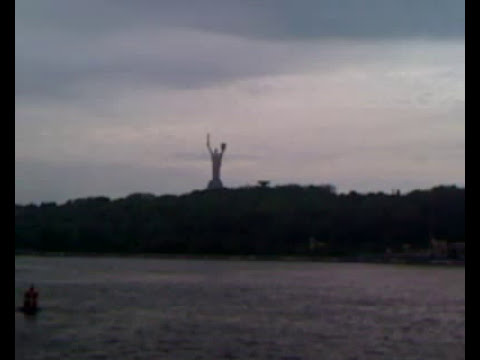In the fuzzy, dark image, a silhouetted scene unfolds with a calm body of water occupying the bottom quarter of the frame. This water, reflecting varying shades of bluish gray, stretches across the foreground, extending into a tree line that spans horizontally from left to right, slightly below the midpoint. Among the dark, nearly black trees, positioned slightly off-center to the left, stands a large, indistinct statue. This statue appears to be holding an object aloft in one hand, with another smaller object in the opposite hand. Above this scene, the upper half of the image is dominated by a sky filled with bluish-gray clouds, adding to the overall somber tone. To the right in the distance, faint outlines of buildings or a settlement can be discerned near the water. Additionally, in the lower-left corner of the water, there is an indistinguishable object—perhaps a buoy or small boat—adding a hint of intrigue to the mysterious landscape.